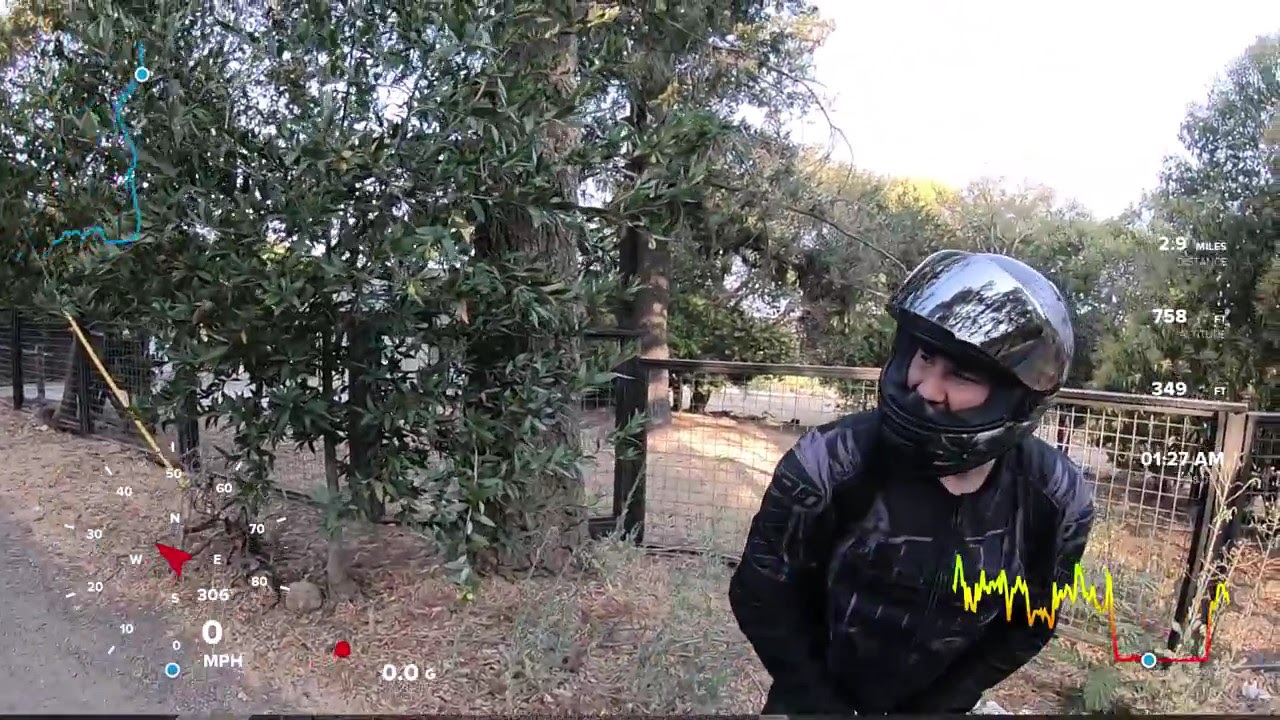In this image, a man dressed in a full motorcycle outfit including a black jacket and a silver helmet with a reflective visor stands facing sideways. He appears ready for motorbike or dirt bike riding. Positioned towards the bottom right of the image, he is framed by a fence with wooden posts that extends into the background. The scene is set outdoors in the daytime, with the sun casting light on the environment. To the left and beyond the fence, there are numerous green trees. The ground beneath him consists of broken-up leaves and patches of grass, some of which appear mostly dead. The sky is bright blue with scattered clouds visible in the upper right corner. Overlaid on the image, in the lower left corner, is a graphic meter ranging from 10 to 80 miles per hour, indicating speed. Additionally, a blue squiggly line resembling a road map is situated in the upper left, and yellow and red squiggly lines are found in the lower right of the image. The overall color palette includes shades of gray, brown, black, white, yellow, orange, red, blue, green, and turquoise.